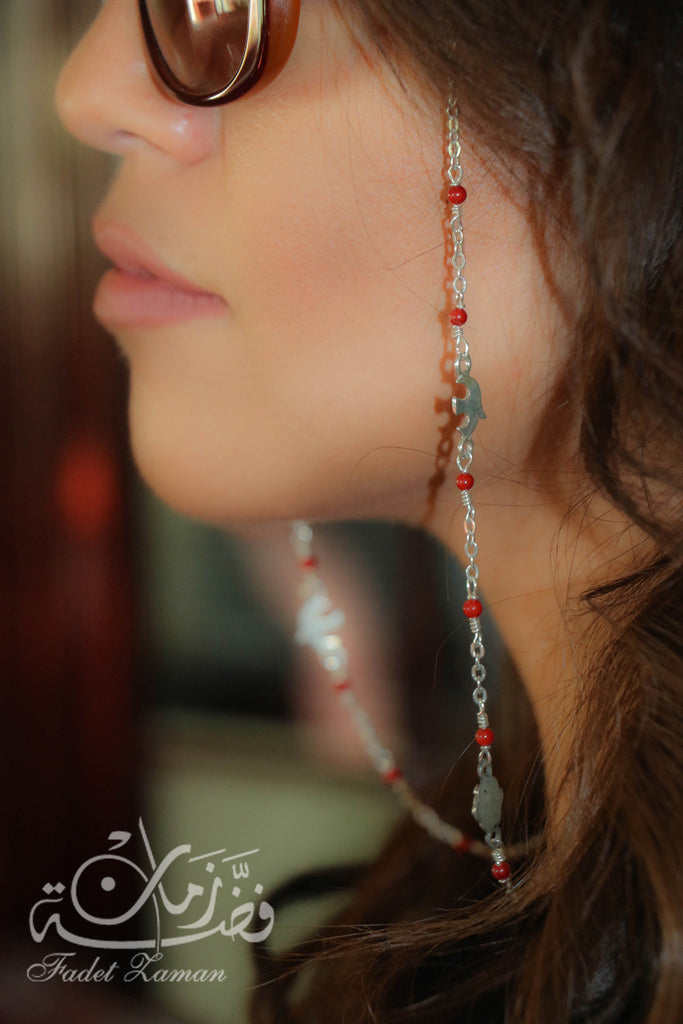This close-up photograph, credited to Fadet Laman with their name written in cursive in the lower left corner, captures a side profile of a young woman in her early to late 20s with dark hair and medium skin tone, looking off to the side. She is wearing dark sunglasses from which hangs a silver eyeglass chain adorned with small red beads and intricate metal animal charms. The chain curves behind her neck, creating a distinctive and stylish look. The background of the image is highly blurred with muted tones of brown, tan, and hints of red, emphasizing the strong depth of field and drawing focus to the subject and the ornate eyeglass chain.